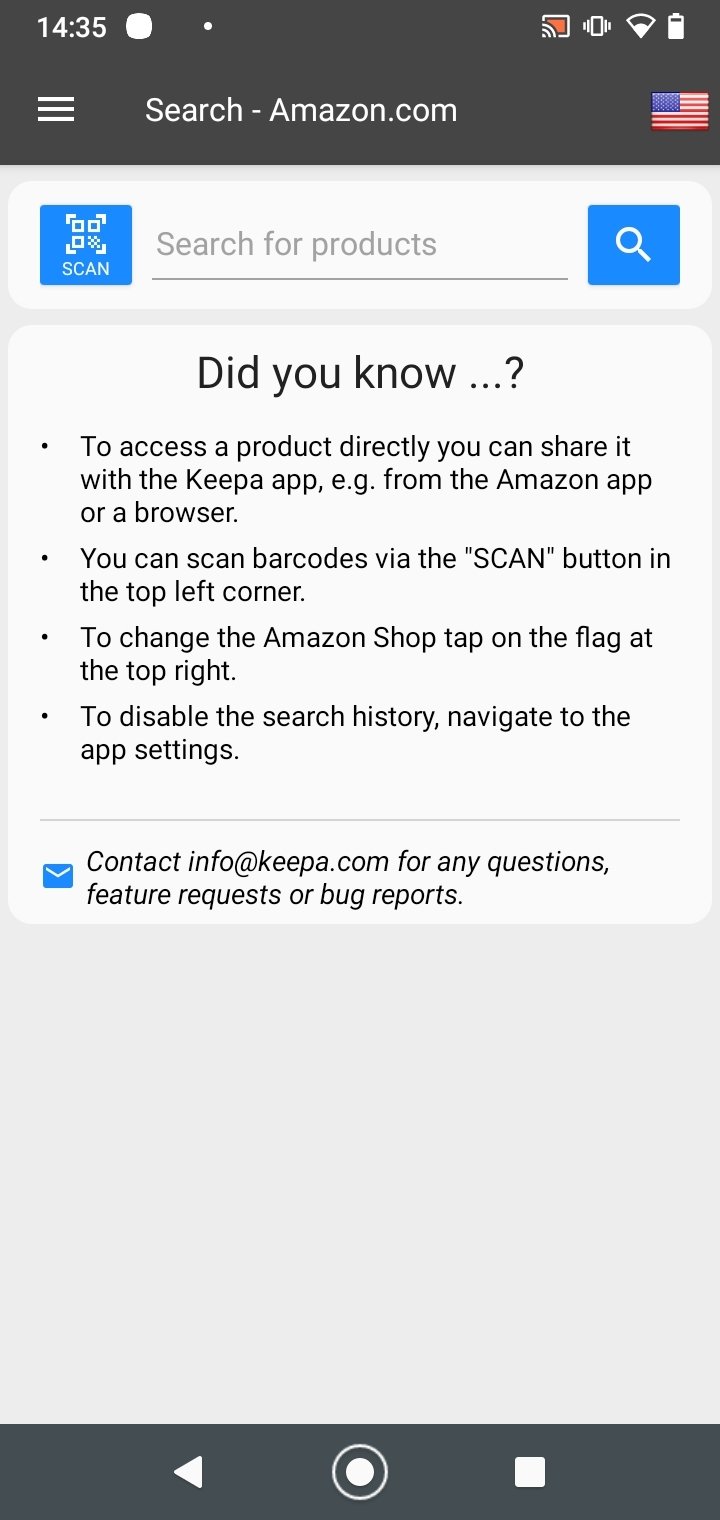The image appears to be a screenshot from a cell phone. At the very top, there is a black border displaying the time in white, "14:35," equivalent to 2:35 PM. A white circle and various status icons - including battery life, Wi-Fi signal, and network signal - appear to the right of the time.

Below this, there are three small white lines adjacent to the text "search-amazon.com." To the right of this URL text is an image of the American flag. The background of this section is grey. 

Towards the left, there is a small blue square labeled "Scan," and in the middle, there's a grey search bar with the text "Search for products" with a grey underline. To its right, there's another small blue square featuring a magnifying glass icon. 

Directly below this search bar, a black text header reads, "Did you know...?" followed by four bullet points in black text:

1. "To access a product directly you can share it with the Keepa app e.g. from the Amazon app or a browser."
2. "You can scan barcodes via the Scan button in the top left corner."
3. "To change the Amazon shop, tap on the flag at the top right."
4. "To disable the search history, navigate to the app settings."

Following these bullet points, there is a grey horizontal line. Below this line, on the left side of the screen, there is a small blue envelope icon. To the right of this envelope icon, text in black reads, "Contact info@keepa.com for any questions, feature requests, or bug reports."